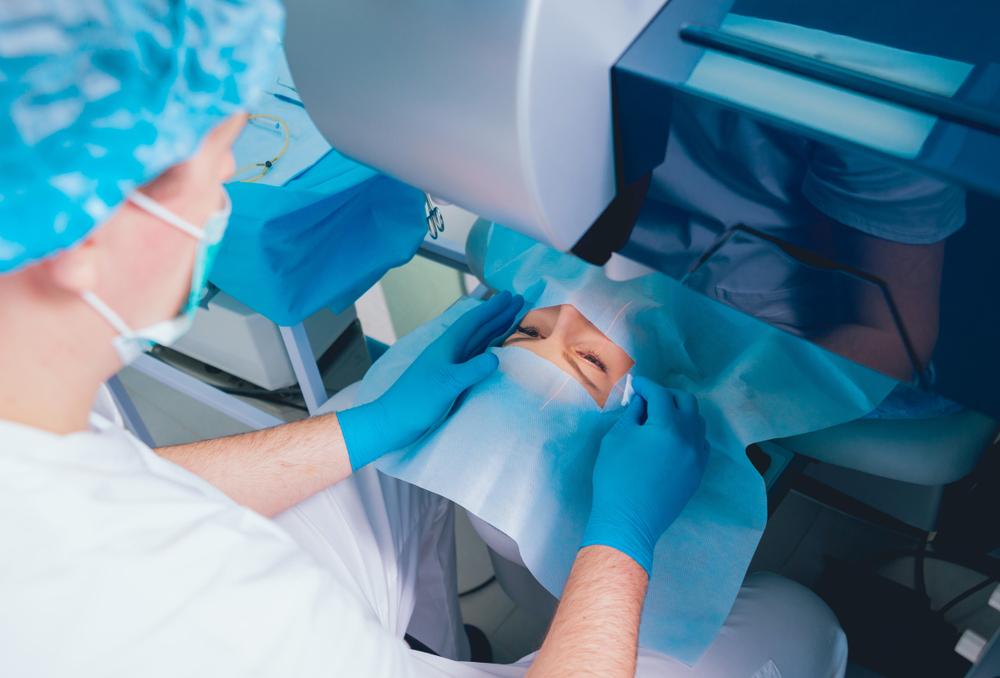In this horizontal rectangular image, a doctor or nurse, identified by a white uniform, blue face mask, and blue cap, is preparing a patient for an eye surgery. The patient is lying face-up with a thin blue drape covering their entire face except for a rectangular area exposing both eyes, eyebrows, and part of the nose. The medical practitioner, wearing blue rubber gloves, is positioned behind the patient's head, holding the drape in place while focusing intently on the patient's face. The setting appears to be a surgical room, indicated by various pieces of equipment in the background, including a gray machine adjacent to the patient, possibly used to stabilize her during the procedure. The reflective surface beneath the patient adds dimension to the sterile environment.